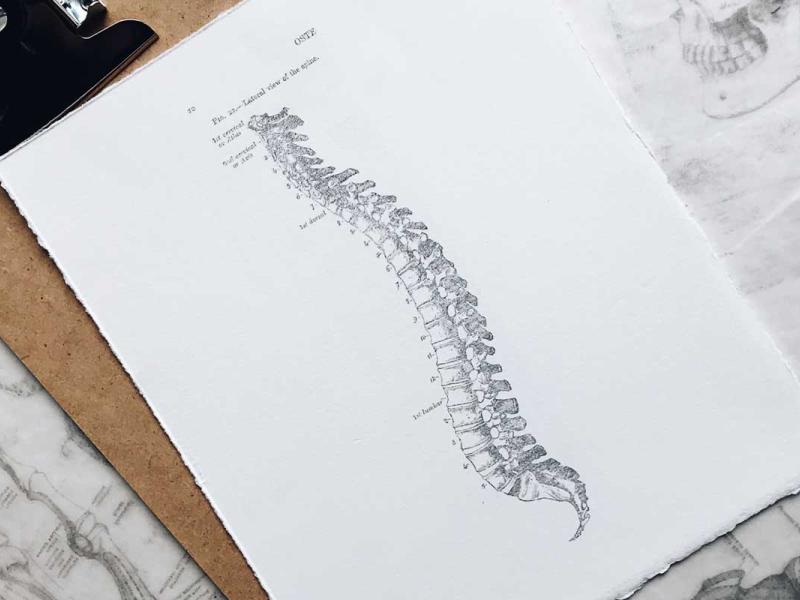The image features a detailed scientific diagram of a spine printed in gray and black ink on a white sheet of paper. The paper is positioned diagonally atop a brown clipboard with a black metal clip at the top. The clipboard, which appears to be made of cardboard or wood, rests on a gray table surface. At the top of the paper, the text "Lateral view of the spine" is visible. The diagram includes various labels identifying different parts of the spine. Additionally, there is a drawing of a skull's mouth and teeth at the top right of the page, along with other anatomical illustrations of body parts and bones located beneath the clipboard. These elements contribute to the detailed and educational nature of the image.